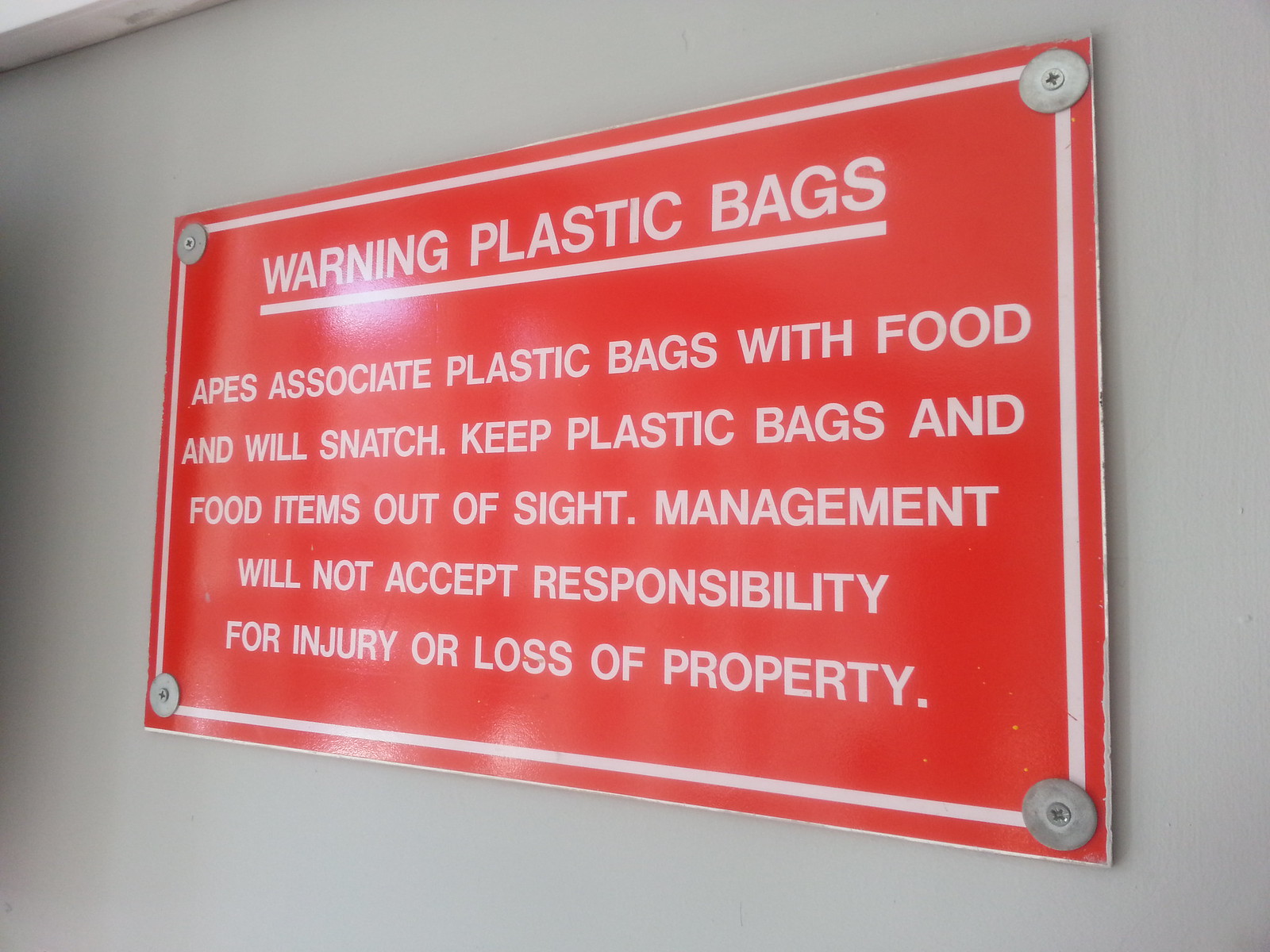This detailed color photograph captures a red, glossy rectangular sign affixed to a light gray wall, with a small portion of the white ceiling visible in the top left corner. The sign's right side is closer to the camera, creating a slightly angled perspective. The sign is secured by wide silver discs, with screws in the center at each of the four corners. A thin white border outlines the sign, which bears white text. At the top, the text "WARNING PLASTIC BAGS" is underlined and in all capitals. Below, the sign reads, "APES ASSOCIATE PLASTIC BAGS WITH FOOD AND WILL SNATCH. KEEP PLASTIC BAGS AND FOOD ITEMS OUT OF SIGHT. MANAGEMENT WILL NOT ACCEPT RESPONSIBILITY FOR INJURY OR LOSS OF PROPERTY," also in all capitals but not underlined. Reflections on the glossy surface create a slight glare, adding a dynamic element to the image. The overall setting suggests the photograph was taken in an indoor environment, possibly a zoo.